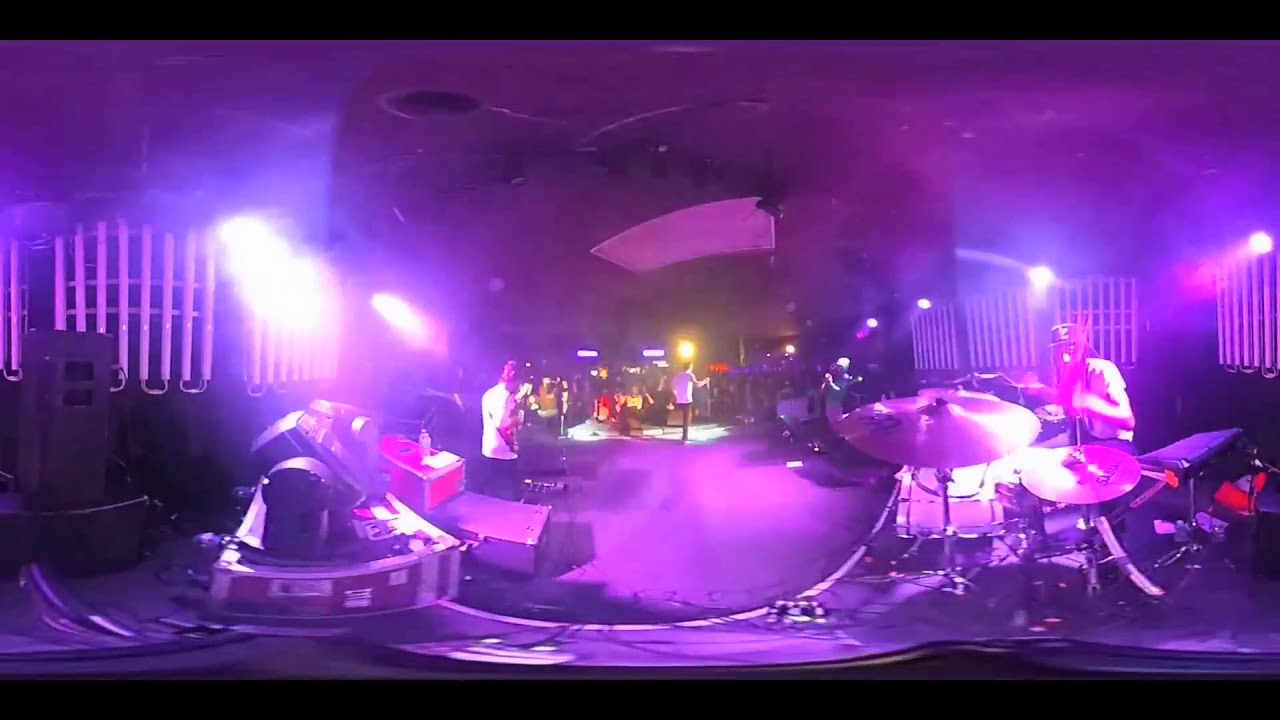The image captures the vibrant scene of a concert stage bathed in dynamic purple and pink lighting. Center stage, a man wearing a white shirt and dark pants stands with one arm outstretched above his head, engaging with the audience. To his right, a bright yellow circle light adds a pop of contrast to the predominantly purple hue. A drummer, positioned on the right side of the image, wearing a white shirt and a black cap, plays behind a white bass drum and two shimmering cymbals. The far left features a white oval-shaped light with paired white tubes hanging against the wall, secured by silver hooks. Below this setup are three stacked boxes in brown, red, and gray. The indoor concert venue is filled with a crowd centrally located, basking in the colorful illumination, making the scene lively and immersive. The overall ambiance is dominated by hues of purple, pink, black, and white, enhancing the electric atmosphere of the performance.